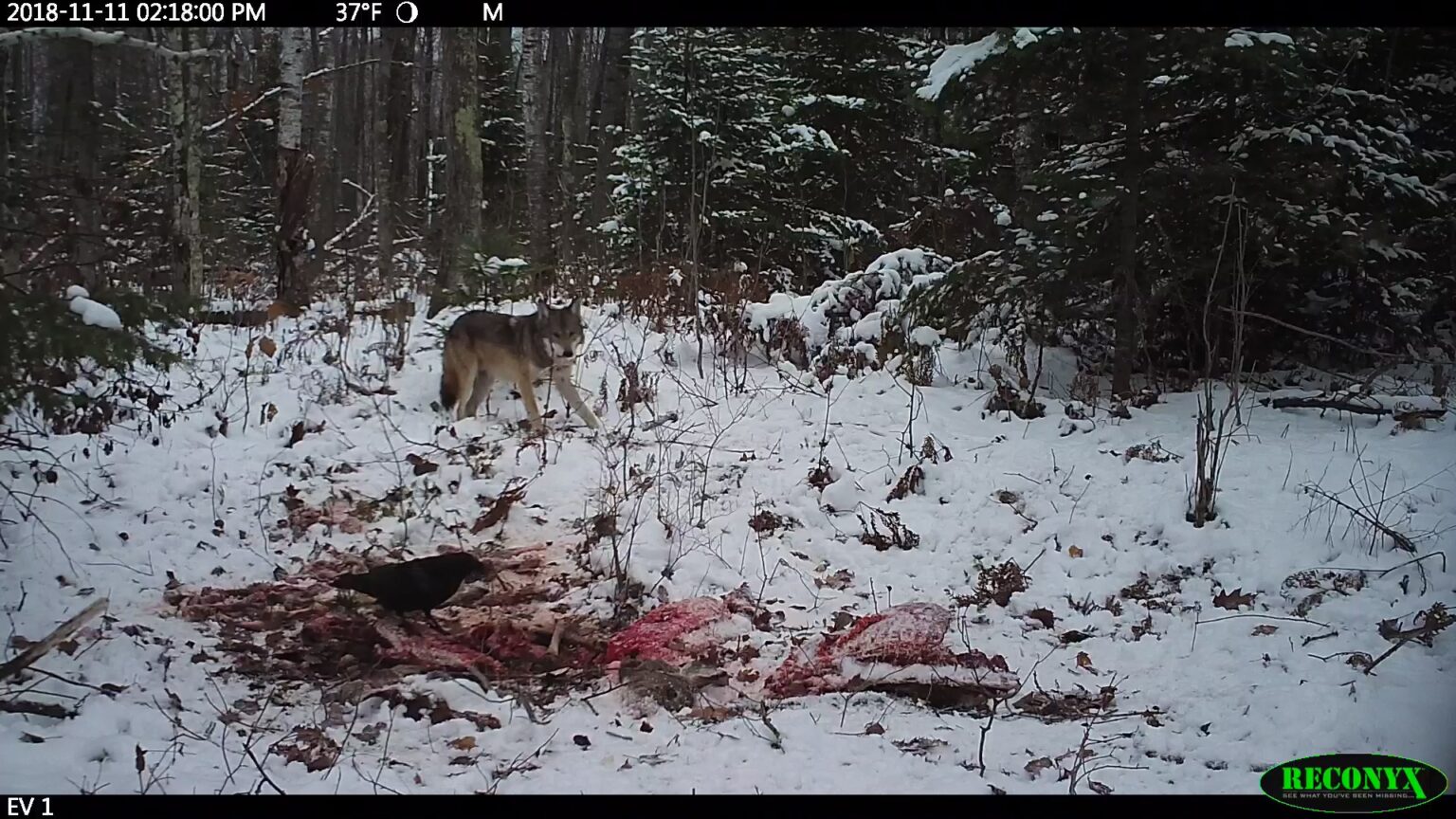An outdoor photograph captured in a snow-covered forest on November 11, 2018, at 2:18 p.m. shows a gray wolf with a white underbelly and gray top walking towards a partially decomposed animal carcass with visible pink flesh. In the foreground, a black crow is perched atop the carcass, pecking at it. The partially snow-covered landscape includes scattered tree trunks and evergreen trees. The image carries the Reconyx logo in bright green text in the bottom right corner, with additional informational text, including the date and time, displayed in white in the upper left corner.